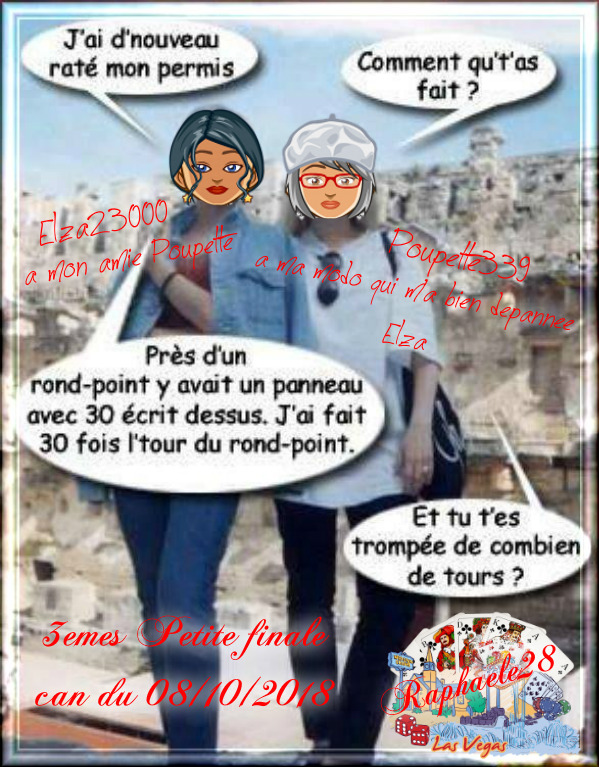This is a colored media print piece from August 10th, 2018, featuring a modified photograph of two women standing in front of an ancient European building, possibly the Colosseum in Rome. While the women's bodies, including their clothes, arms, and necks, are actual photographs, their faces have been replaced with cartoon-like ink drawings, giving the entire image a composite and somewhat whimsical appearance. The woman on the left, dressed in a white t-shirt and dark blue or black jeans, has lighter hair, wears a white beret and red glasses, and carries a dark blue handbag. The woman on the right is in a jean jacket and jeans and has darker hair with earrings. Both women are engaged in a conversation in French, with speech bubbles over their heads. The dialogue reads:

Left Woman: "Comment que t'as fait?" (How did you do it?)
Right Woman: "J'ai de nouveau raté mon permis." (I failed my driving test again.)

In a continuation:
Right Woman: "Près d'un rond-point il y avait un panneau avec 30 écrits dessus. J'ai fait 30 fois le tour du rond-point." (Near a roundabout, there was a sign with '30' written on it. I went around the roundabout 30 times.)
Left Woman: "Et tu t'es trompé de combien de tours?" (And how many times did you get it wrong?)

The piece includes a number, "ELSA 23000," on the left-hand side, and a text at the bottom stating "3ème Petit Finale Condu, 8-10-2018" and "Raphael, 28, Las Vegas."